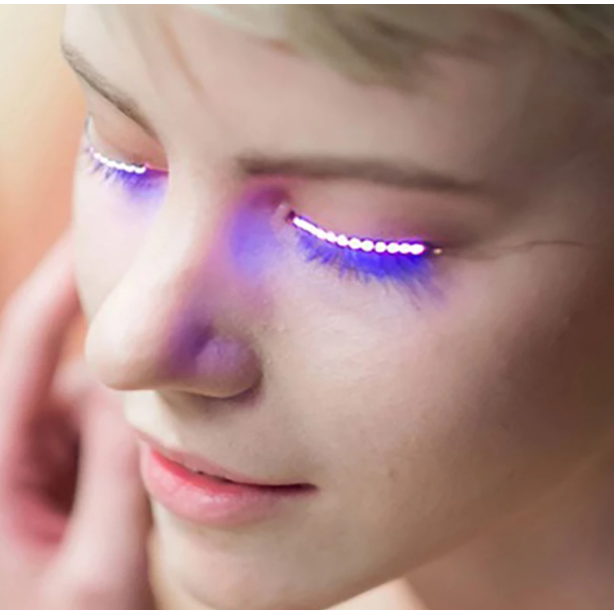This close-up image captures the face of a blonde Caucasian woman in her early 20s, positioned with her nose directed slightly to the left of the frame. The camera angle is from above and to the front, giving a dynamic view of her pale white skin and light brown hair that peeks into the top right corner. The most striking feature of this photograph is her unique, illuminated eyelashes. The eyelashes themselves appear natural, but they are adorned with numerous tiny LEDs along the base, emitting a vibrant neon blue light. These LED lights create an effect similar to sequins or rhinestones, distinctly visible where the lashes connect to her eyelids. A slender wire, likely connected to a concealed battery pack, can be seen extending from the edge of her eyelid when viewed from the top left. Additionally, her hand gently touches the right side of her face, adding a subtle, blurred element against the otherwise sharply focused background.